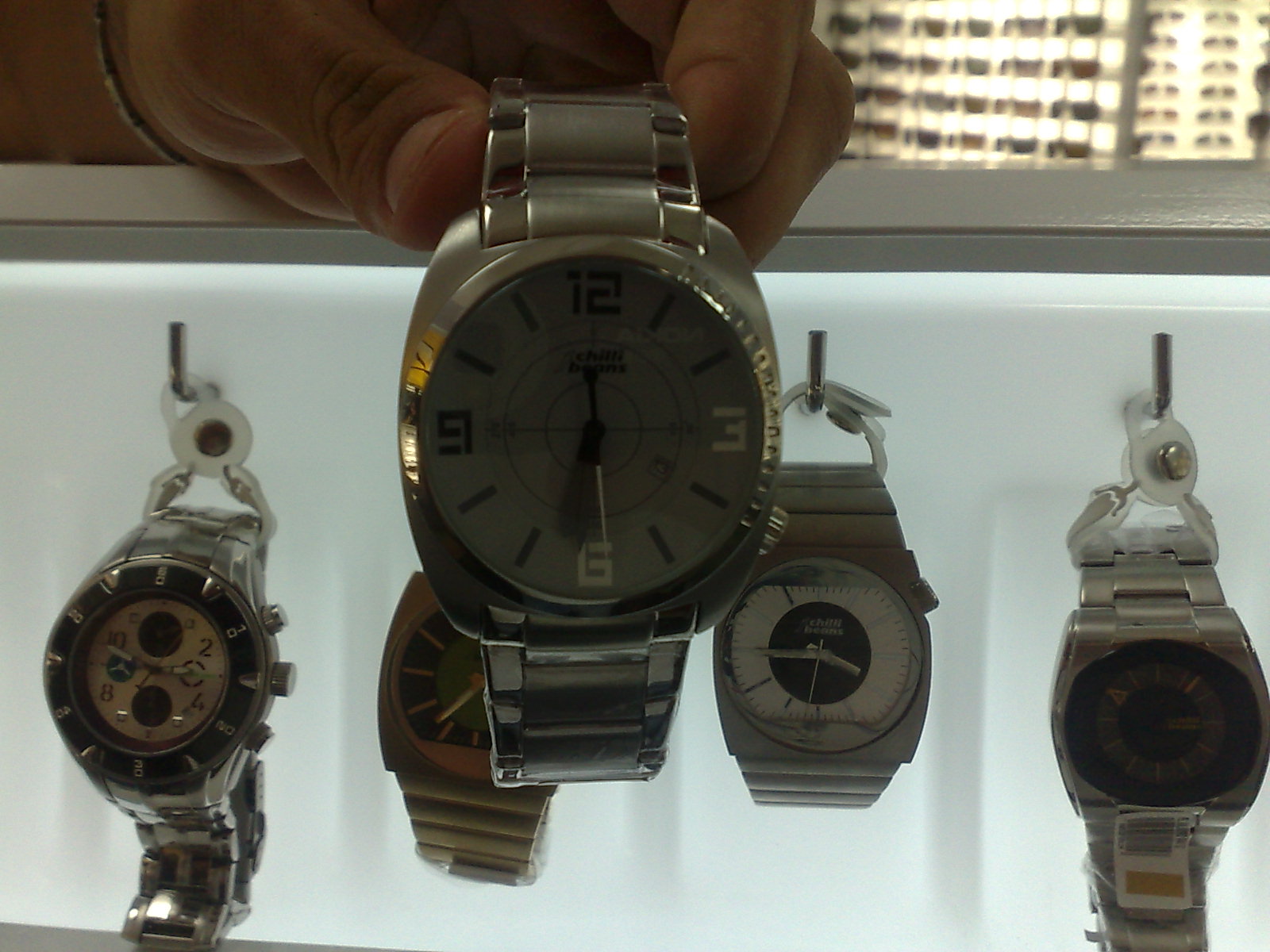A close-up photograph showcases a man's hand holding a silver watch against a backdrop of additional silver men's watches, all displayed in a case. The held watch indicates a time of approximately 6:30 or 6:32. Other visible watches display times of around quarter to four or quarter to three. The man's hand, with thick fingers and a bracelet on the wrist, rests on a counter as it secures the watch. In the background, a lit-up display case of sunglasses can be seen, with the illuminated wall casting a white glow and highlighting the distinct shapes of the eyewear.